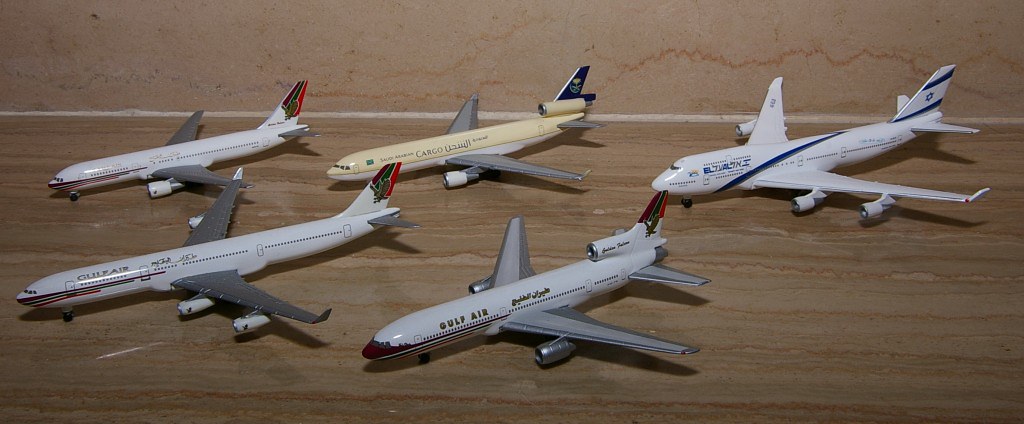This photograph depicts a collection of five meticulously crafted model airplanes, each representing various civilian airliners, displayed on a wooden countertop against a peach-colored wall with accents of brown, blue, and purple. Prominently featured in the center of the arrangement is a white Gulf Air model with dark gray wings and white engines on either side, accentuated by golden cursive writing. To its left sits a striking beige plane with a white underside and gray wings, marked "cargo." Above it, another Gulf Air model stands out with light gray wings, a black nose, and a secondary engine near its tail fin. On the far left, a plane adorned with red and blue stripes suggests it hails from the same manufacturer. In the background, an imposing white aircraft with a blue line and an Israeli flag on its tail fin completes the ensemble. The wall behind the planes has a water-stained texture, enhancing the display's intricate and personal feel.